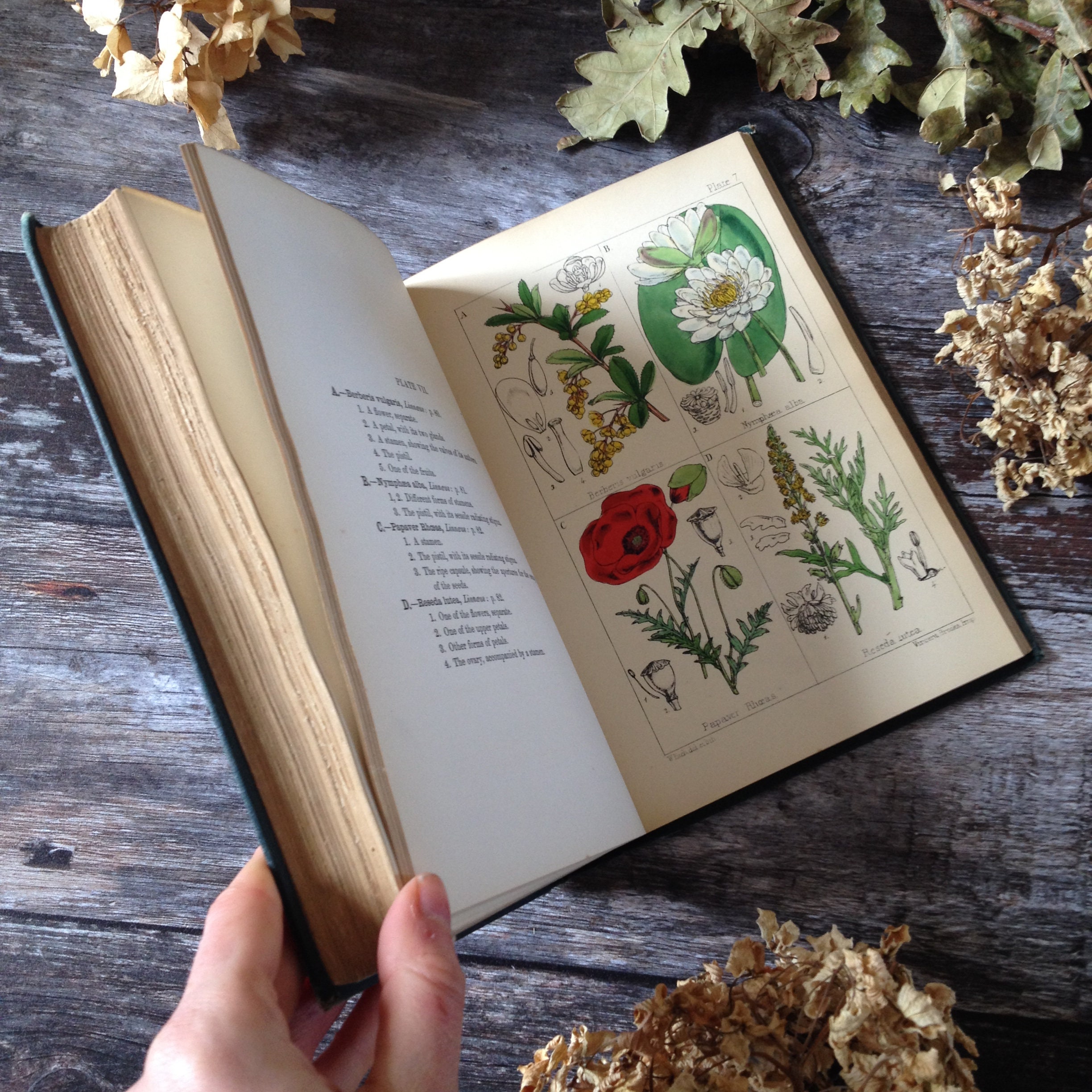The image features a meticulously staged scene akin to a curated Instagram photo. At the heart of the image is a hand with lighter skin, prominently holding open a blue hardcover book that appears aged and worn. The focal point of the open pages presents a pictorial guide to flowers: a white flower with a yellow center, possibly a daisy, and a red, fully open flower, perhaps a rose. The left page contains black text, resembling a quiz or chart with listed facts beneath several headings. Surrounding the book is a weathered, dark gray wooden table or plank, enhanced by a deliberate arrangement of both dried and green leaves. The distressed wood adds a rustic charm, while the mix of dead flowers and live leaves framing the top left, upper right, and bottom of the image creates an atmosphere of juxtaposed life cycles. The setting is brightly lit, ensuring all details are captured with clarity and sharpness.